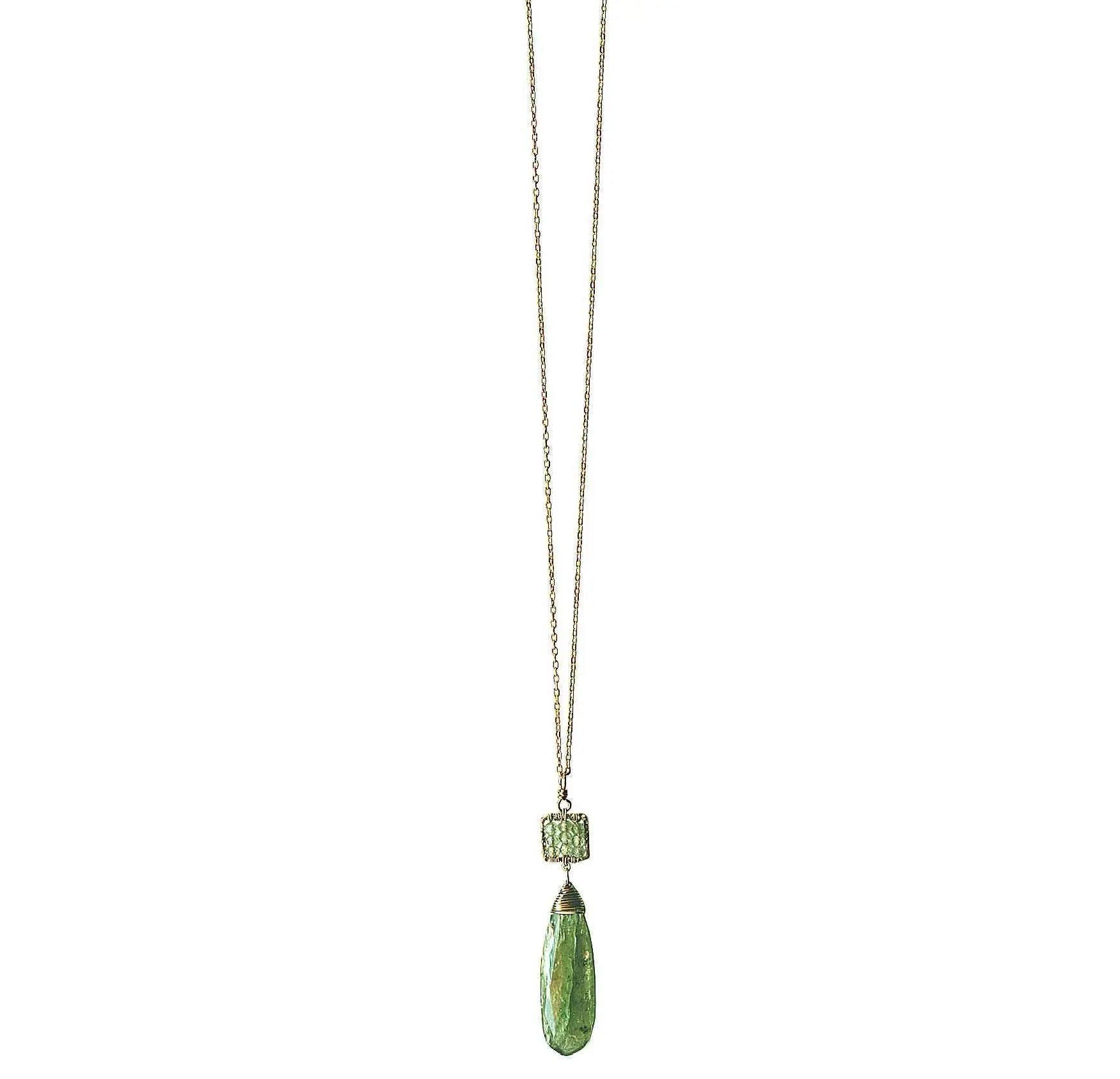The photograph features a delicate necklace prominently displayed against an immaculate white background, creating the illusion of the piece floating in a void. This minimalist setup emphasizes the product, ideal for online commercial purposes. The necklace showcases a slender, finely-linked gold chain that extends from the top edge of the image, partially cut off, creating a seamless look. The meticulously crafted links are small and intricate, highlighting the necklace's elegance.

Suspended from the chain is a silver ring that connects to a distinctive pendant. The pendant begins with a light green, square-shaped stone encased in an ornate metal netting, adding an element of sophistication. Beneath this stone, a smaller chain segment leads to a secondary pendant: an elongated, oval-shaped green gemstone. This lower gem is capped with a polished silver tip, completing the pendant's design. The combination of the square and oval green stones, along with the intricate chain work, makes for a striking and elegant piece of jewelry.